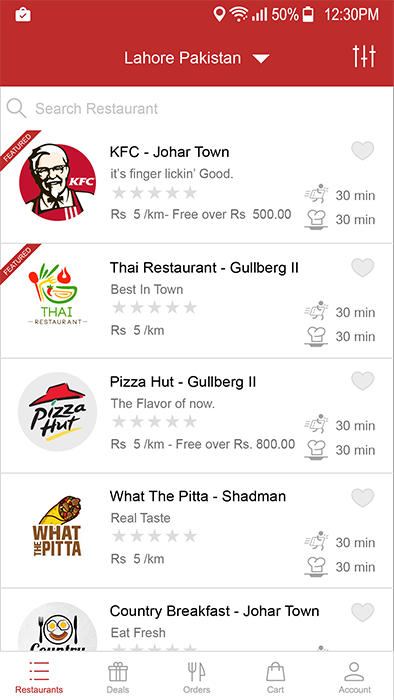The image captured from a person's phone screen showcases various dining options they were considering in Lahore, Pakistan. The top of the screen features a red banner with white text that reads "Lahore, Pakistan." Beneath the banner, there's a search bar with a magnifying glass icon labeled "Search Restaurant." 

The first listing prominently displayed is for "KFC Johar Town," marked as "Featured" in a banner, with the iconic Colonel Sanders logo and tagline "It's finger-licking good." The distance indicated is "5 kilometers." 

Following this is "Thai Restaurant Goldberg 2," also marked as "Featured" with a corresponding banner and an icon on the left side. It’s described as the "best in town" and is located 5 kilometers away. 

Further down the list, other dining options include "Pizza Hut," "What the Pita Shadman," and "Country Breakfast Johar Town," each with their respective icons and details.